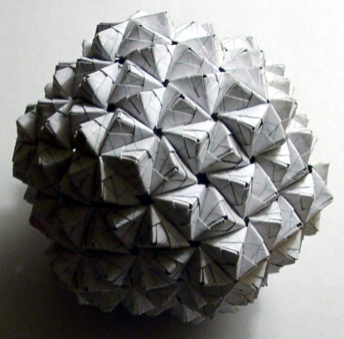This square-shaped photograph captures a round object intricately covered in a myriad of triangle-shaped facets, creating a textured pattern across its surface. The object is predominantly white, accentuated by dark gray lines that define the edges of each triangle, contributing to a distinctive geometric appearance. The background of the image is light gray, providing a neutral canvas that enhances the visual prominence of the spherical subject. A noticeable shadow is cast on the bottom left corner, adding depth and dimension to the composition, suggesting that the illumination originates from the upper right, highlighting that side of the object and creating a striking contrast across its form.